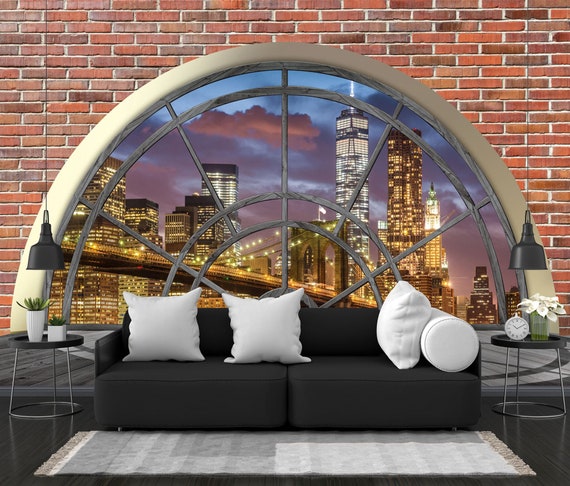The image is a highly detailed indoor scene, likely an artist's illustration of a luxurious living space. The backdrop features an exposed red brick wall dominated by a large, arched half-circle window with white borders and a spider-web-like gray pane design. Through the window, the evening sky is tinged with purplish hues, revealing a brightly lit cityscape with prominent skyscrapers and the Brooklyn Bridge, one building showcasing an illuminated American flag.

In front of the grand window stands a modern black sofa adorned with three white square pillows and one cylindrical white pillow. Flanking the sofa are two black circular side tables, each with stainless steel legs arranged in a circle. The table on the left holds two potted succulents in white ceramic pots, while the right table features a white clock and a green vase with white lilies.

Above each table hangs a black pendant lamp with a black cord. The scene is anchored by a gray and white striped rug with tasseled edges on each end, covering the gray hardwood floors, adding to the room's sophisticated ambiance.